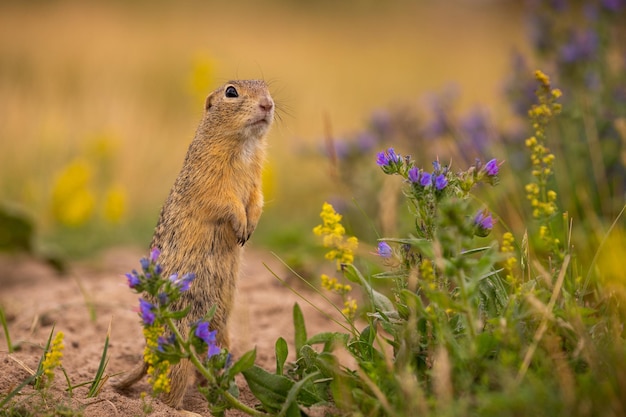This detailed photograph captures a prairie dog standing upright on a dirt path amidst a setting of wildflowers and grass. The prairie dog's front paws are together in front of its stomach, and it has an alert expression, gazing off to the left as if sensing something. The vivid scene includes clusters of purple and yellow flowers that are roughly the height of the prairie dog, adding pops of color to the foreground. The background of the photograph is artistically blurred, ensuring the prairie dog and the surrounding blooms remain the focal point. The well-composed image provides an intimate, ground-level view that captures the natural beauty and keen vigilance of the prairie dog in its habitat. The prairie dog’s one visible eye and the positioning of its small, curled front paws contribute to its apprehensive appearance, adding a layer of narrative to this captivating nature shot.